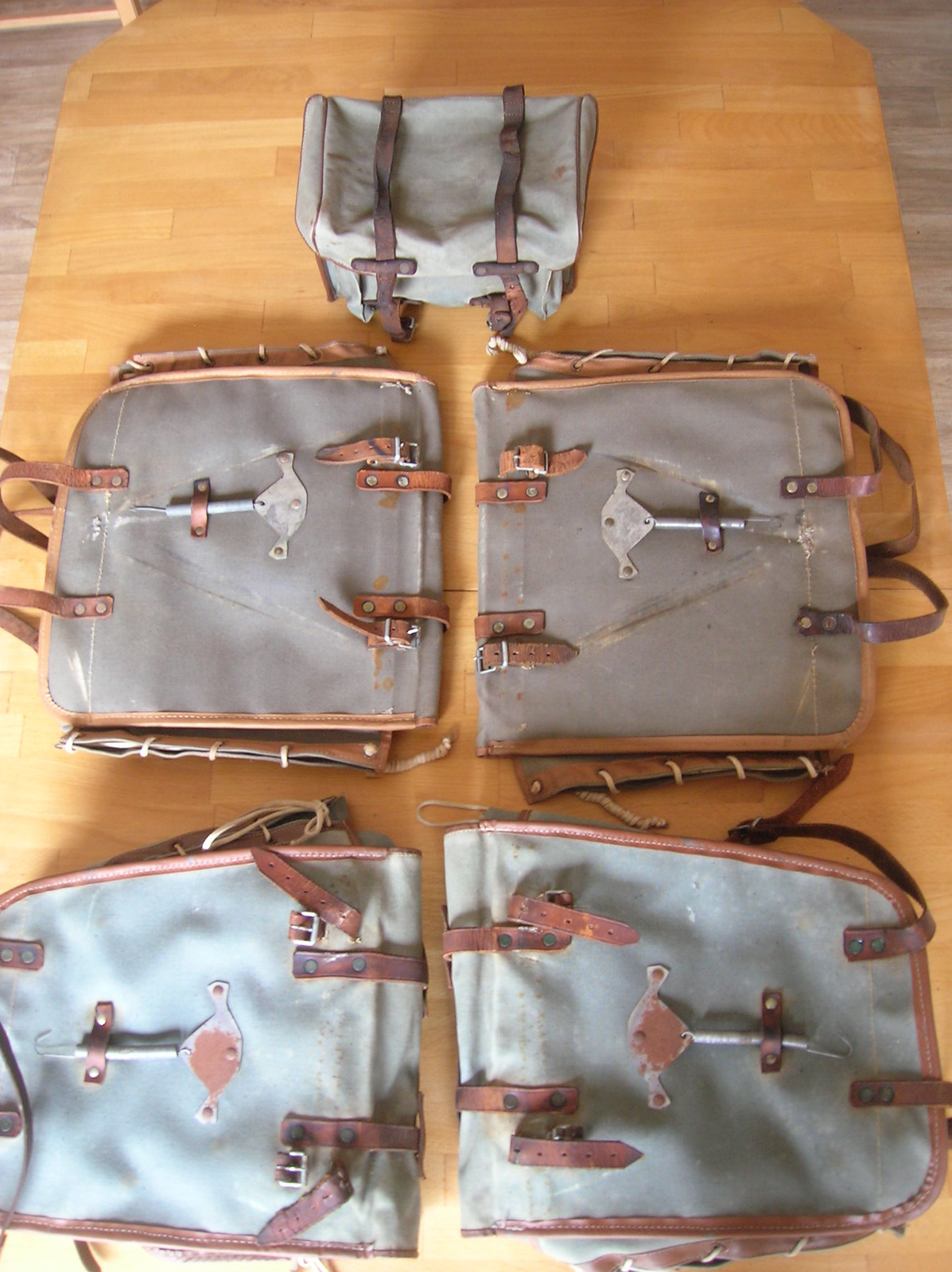This image is a detailed overhead shot of five gray tote bags with brown leather straps, arranged on a light brown wooden surface. Four of the bags are larger and similarly designed, with brown straps and a metal piece attached via a loop, giving them a slightly antiquated look. These larger bags are arranged in two pairs, with each pair featuring a slightly different shape—one pair being more rectangular and the other a bit narrower and longer. The smaller bag in the center, resembling a lunchbox in shape, also has the same gray color and brown straps as the larger ones. The light brown wooden surface adds a warm contrast to the gray and brown tones of the bags. The setup appears intentionally organized, with the two pairs of large bags lying flat and facing each other, while the smaller, rectangular bag is positioned above them, completing the symmetrical arrangement.